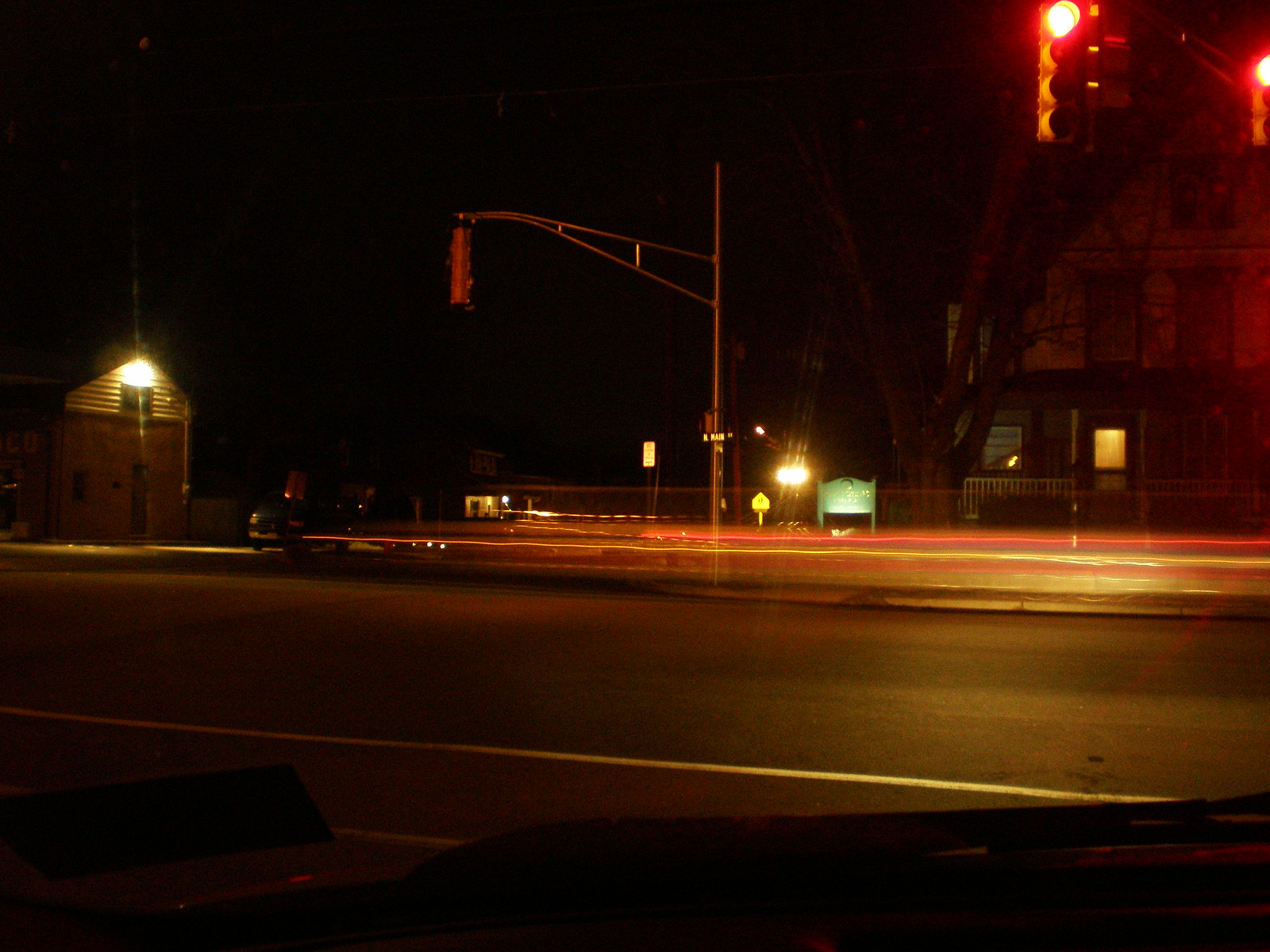A nighttime photograph captures a bustling street intersection. The road, clearly marked with yellow lines down the center, leads the eye towards a scene of urban activity. On the left, a building illuminated by a regular exterior light stands prominently. Streetlights punctuate the scene, with one facing away from us and another glowing red in our direction. 

Behind the traffic lights, a structure that resembles a house but features a sign hints at a potential business or public building. Blurred cars streak past, adding dynamic movement to the scene. The headlights of a distant vehicle pierce the darkness, contributing to the lively and somewhat mysterious nighttime atmosphere.